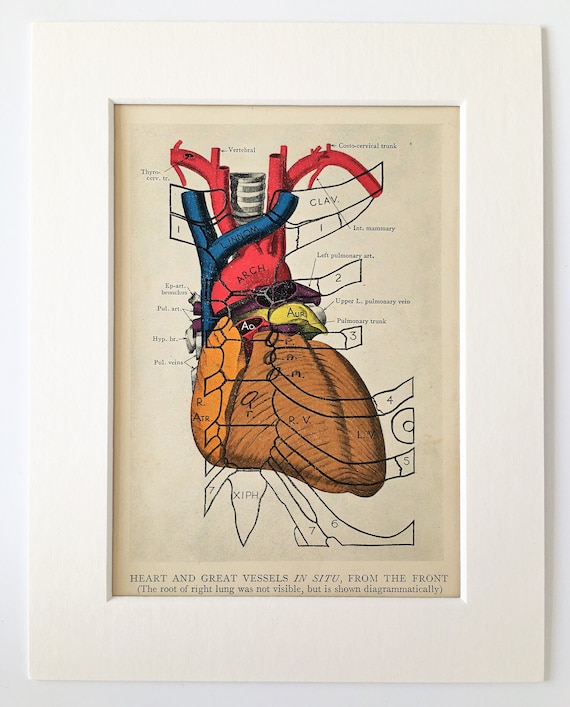This detailed anatomical illustration depicts the human heart and its great vessels in situ from a front view, rendered in vivid colors and framed by a light or off-white art mat. The heart is meticulously color-coded to differentiate between oxygenated and deoxygenated blood pathways: red denotes oxygenated blood pathways, while blue represents deoxygenated ones. Yellow shading highlights the atria, whereas brown is used for various other sections of the heart. The illustration is annotated with detailed labels and abbreviations, such as RV for the right ventricle, each accompanied by explanatory notes. Additionally, arrows point to specific parts, including an arrow indicating the left pulmonary artery. The illustration is produced on a background that appears aged, with a slight yellowish tint suggesting it is over a century old. Text at the bottom clarifies the perspective of the illustration, noting that it provides a front view of the heart and great vessels and includes a diagrammatic representation of the right lung, which is otherwise not visible.